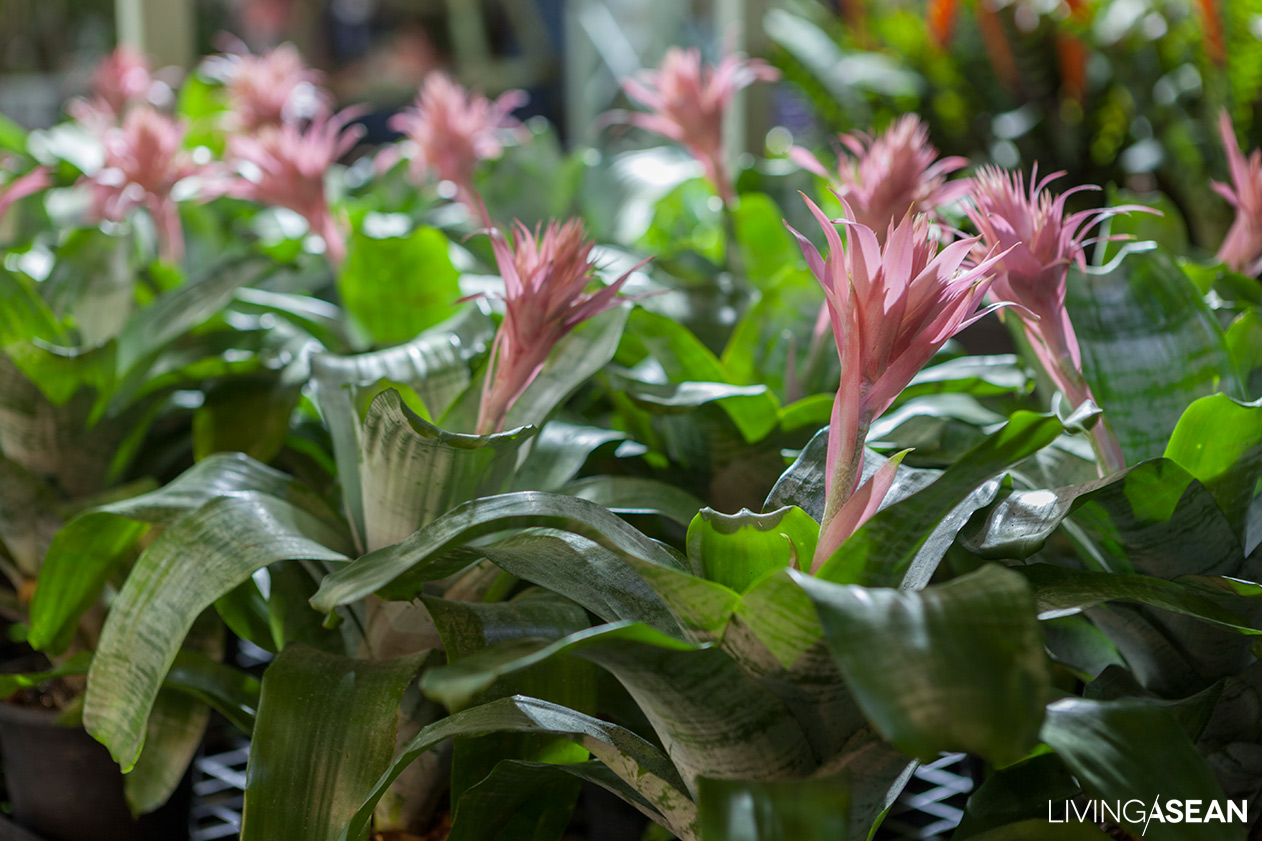The image captures a bright, sunny day in an outdoor setting, possibly a nursery, with a line of bromeliads arranged on a table, each showcased in individual pots. The main focus prominently features the first three bromeliads in the foreground, displaying their striking pink flower buds emerging from the center of their long, broad, and glossy green leaves with white undersides. These tongue-like leaves converge to highlight the slender pink stalks topped with feathery flower buds. The background, slightly blurred, suggests additional rows of similar plants, along with some indistinct flower varieties or possibly different plants. Shelves and gardening equipment are faintly visible, adding to the scene's immersive nursery ambiance. In the bottom right corner, the logo "Living Eshan" is clearly displayed in white text, grounding the photo with its subtle branding.